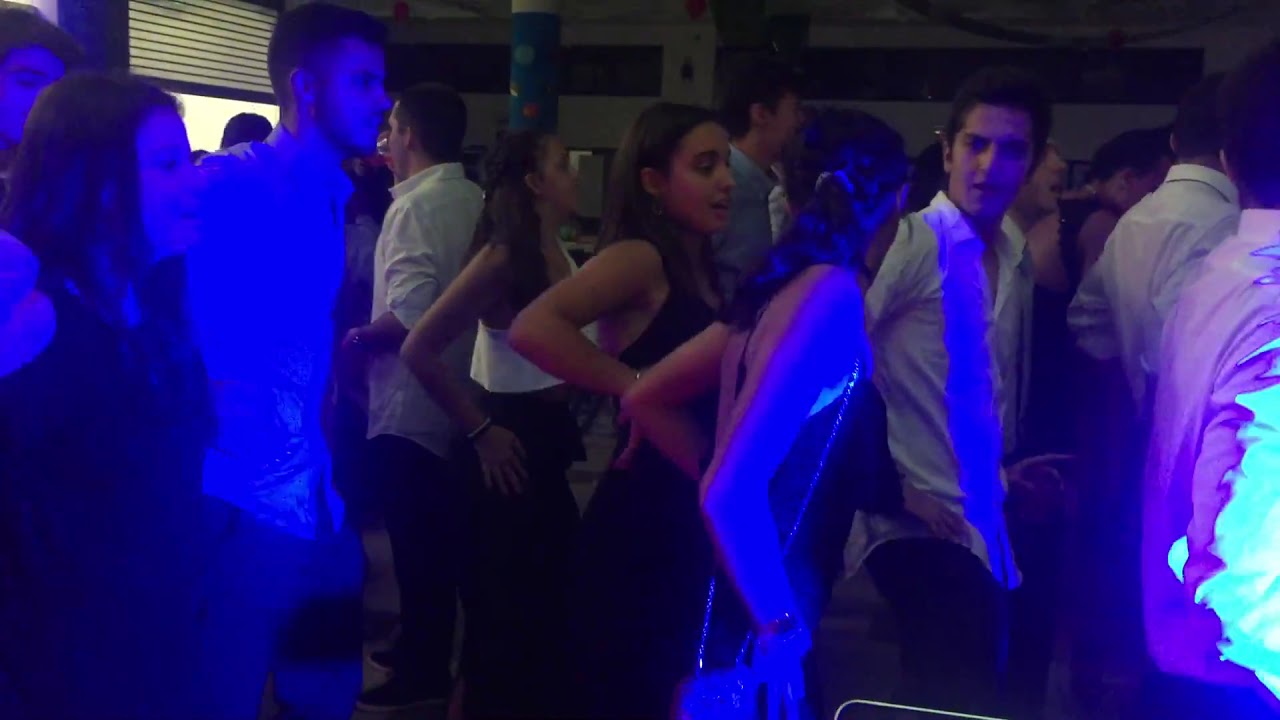The image captures a lively and vibrant gathering that appears to be an indoor party or dance, possibly an office event, adult prom, or nightclub. The room is filled predominantly with young adults likely in their 20s, and a few in their early 30s, dressed elegantly in white shirts and black dresses. The setting is mostly dark with blue lighting creating a nightclub-like ambiance. 

A partially open window with blinds on the left side of the image allows some daylight to pierce through, contrasting with the dim interior. In the background, a large group of young adults is gathered, many facing forward and seemingly engaged with a screen that emits light, though the screen itself isn't visible in the image. There's an air of excitement as some appear to be singing with their mouths open and hands on their hips, suggesting they might be dancing or enthusiastically enjoying a performance. 

One notable couple on the left appears to be in a heated discussion or possibly dancing closely, with the man looking exasperated. Above them, someone is seen drinking, adding to the festive atmosphere. The overall scene is one of vibrant energy, with everyone vibing and living it up, making it a unique and fun moment captured in time.